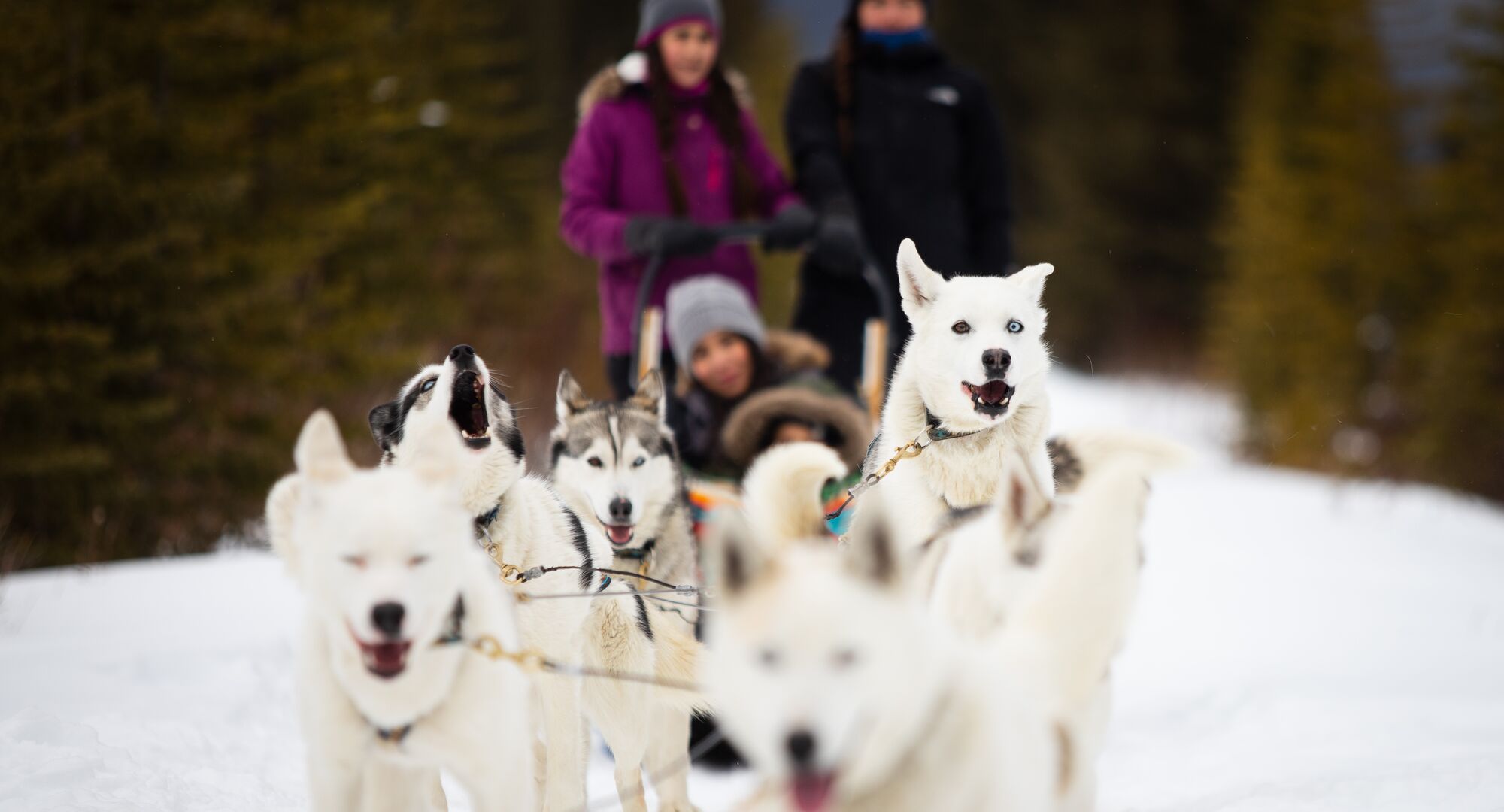In a snowy forest adorned with towering evergreen trees, a dynamic scene unfolds featuring a dog sled team of six energetic huskies with striking blue eyes and varied fur patterns, including white, black, and brown. The sled, driven by a woman wearing a distinctive magenta-purple jacket and a gray toboggan, cuts through the pristine snow. In the sled, another woman, characterized by her brunette hair and black jacket, sits beside a small child bundled in a furry hooded coat. A third person, gender ambiguous due to their all-black attire with a hint of blue, stands to the right. The huskies, some caught mid-howling, appear enthusiastic and spirited as they pull the sled, their expressions reflecting a deep engagement with the task. The image captures a moment of adventure and connection between humans and their loyal sled dogs amidst the tranquil beauty of the winter landscape.